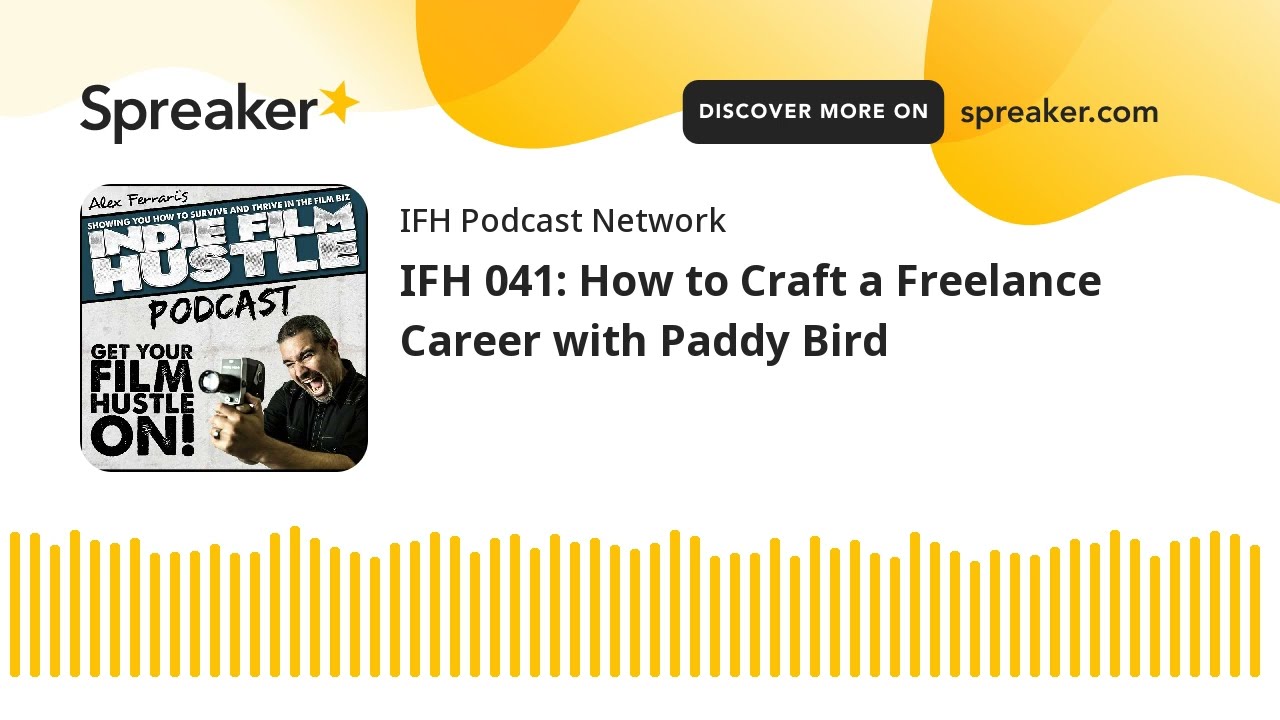The advertisement is for the Indie Film Hustle Podcast on Spreaker. It's set against a primarily white background. At the very top, there are curved yellow designs with text in black reading "discover more on Spreaker.com" on the upper right, alongside the word "Spreaker" with a five-point yellow star next to it on the upper left. 

In the center, there's another yellow banner with the text "IFH Podcast Network" in black. Below this, in similar black text, it reads "IFH041: How to Craft a Freelance Career with Patty Bird." To the left of this text block is a gray avatar graphic labeled "Alex Ferrari's Indie Film Hustle Podcast." Below that, in the lower-left corner, it says "Get Your Film Hustle On!"

The bottom section of the advertisement features vertical yellow bars depicting a sound wave. 

Additionally, the lower right of the central graphic showcases a man appearing excited, holding an old-school movie camera, amplifying the dynamic and engaging theme of the podcast as he seems to be yelling at the camera, aiming to capture the viewer's attention.